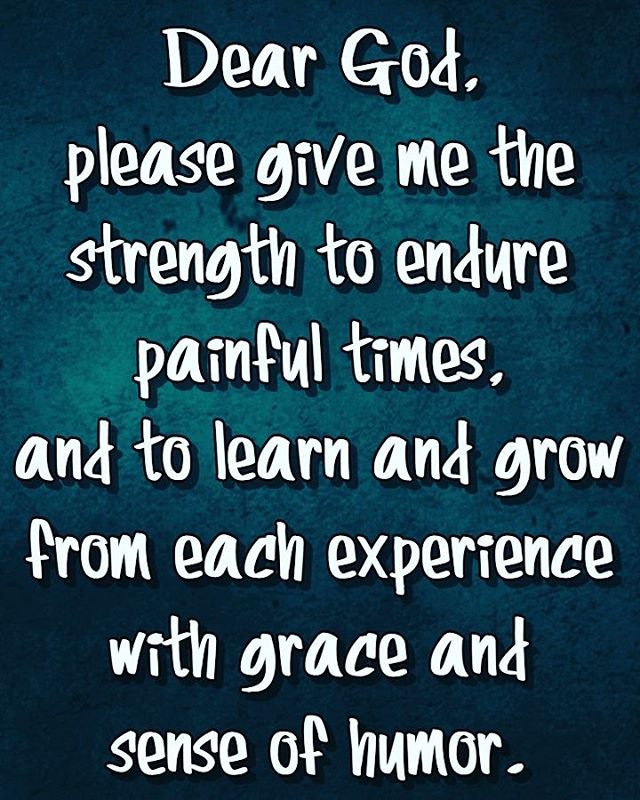This is an abstract, vertically-oriented, motivational graphic art piece featuring a heartfelt prayer. The text, in a bold, bubbly, handwritten-style white font, reads: "Dear God, please give me the strength to endure painful times and to learn and grow from each experience with grace and a sense of humor." The background is a rich, dark blue that lightens slightly toward the top, blending with hints of green to create a dynamic, multicolored effect. Accentuated by subtle, darker blue dots and lines, the background offers a textured and flowing appearance. Overall, it's a soothing and uplifting visual reminder of resilience and grace.